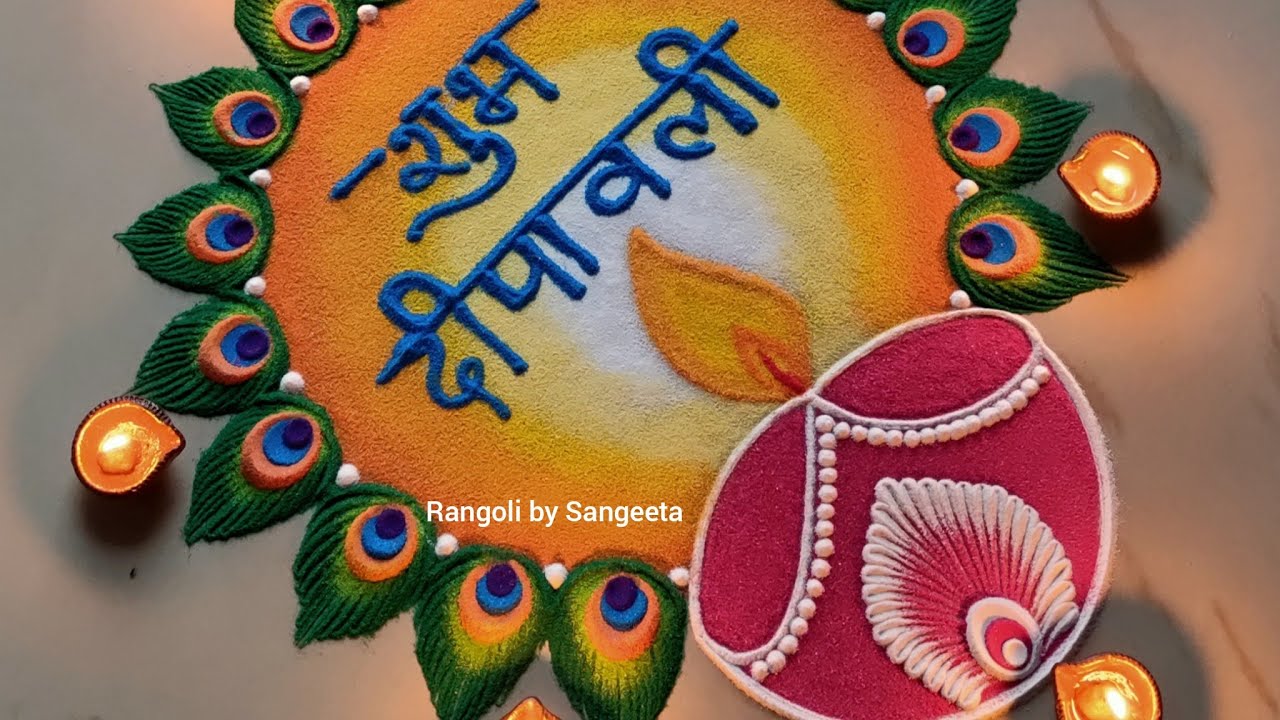This image is a vibrant and intricate piece of decorative art, likely a traditional Indian rangoli, created with what appears to be fabric, felt, or sand. The design features a large circular motif with an orange gradient background that simulates the warm glow of a candle's aura, starting with lighter orange at the center and transitioning to darker orange at the edges. At the center of the circle is a pink candle with white details and a stylized flame made from felt or cloth. The candle is adorned with white pearls and a detailed peacock feather pattern.

Surrounding the central candle are smaller, vivid green peacock feathers, each intricately detailed with concentric ovals in shades of orange, blue, and dark tones. Above the candle, there is blue text in Hindi, which adds cultural significance to the artwork. The entire piece is positioned diagonally on a light-colored surface, accentuating its visual impact.

Additionally, the art is framed by four lit candles in cylindrical holders, positioned around the outer edges of the rangoli, further enhancing the aesthetic appeal and suggesting a ceremonial or festive context. The text "Rangoli by Sangeeta" is prominently displayed at the bottom of the image in white letters, attributing the beautiful creation to its artist, Sangeeta.